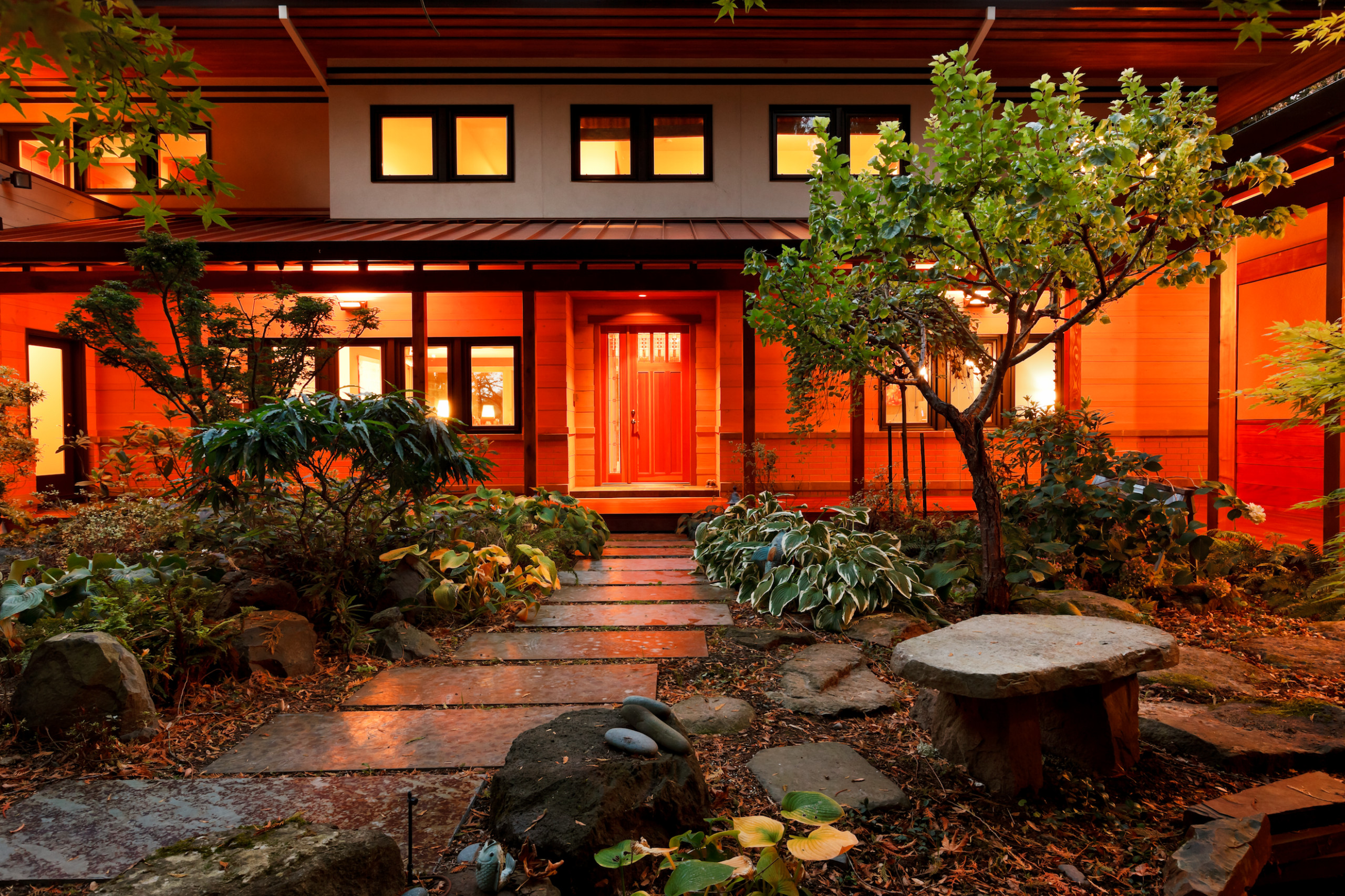The image captures a serene, Asian-style garden set before a two-story house-like structure, photographed at night in landscape orientation. The courtyard features an array of lush greenery and shrubbery on both sides, with scattered leaves adding to the natural ambiance. Large rectangular stone pavers create a pathway leading to a central brown door, which has clear glass panels and is framed by multiple windows above and around it. Soft, warm lighting from the porch's roof and additional fixtures on the walls bathes the entrance area in a reddish-orange glow. The house exterior, which appears to combine wood panels and possibly stone, is complemented by brown vertical supports holding up the roof. On the right side of the garden, a stone platform functions as a bench next to a tree, offering a peaceful spot to sit. The garden is enclosed by reddish walls, suggesting an indoor setting, such as within a hotel or mansion, that maintains a tranquil, relaxing atmosphere despite the nighttime backdrop.